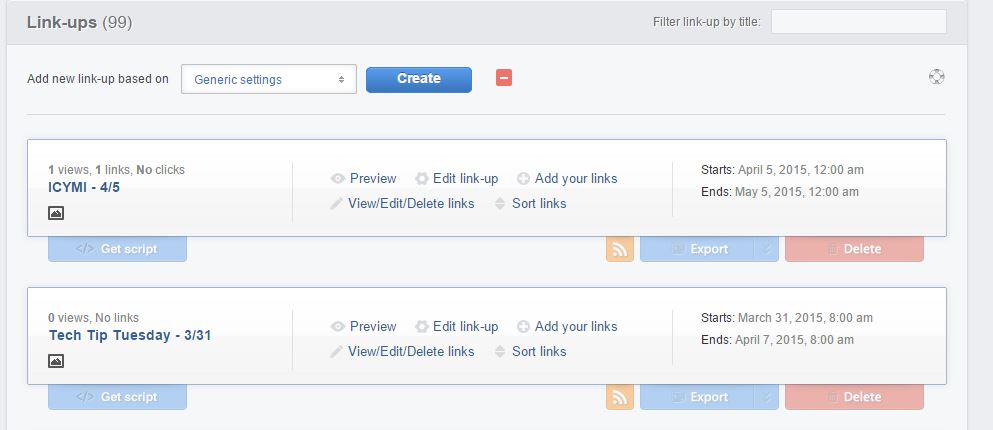This image depicts a detailed settings page designed for managing "Link-ups." The layout is as follows:

At the top of the page, a dark grey bezel provides a clean separation. On the left-hand side, the label "Link-ups (99)" is prominently displayed in black text. On the right-hand side, users are presented with an option to "Filter link-ups by title," adjacent to which is a light grey, clear rectangular search bar.

Below that, the option to "Add new link-up based on" is provided with a light grey rectangle featuring blue text reading "Generic settings" and two black arrows indicating up and down navigation. Next to this, a dark blue button with bold white text reads "Create." Following this, an orange square with a white line through it is displayed alongside a new light grey rectangle.

Within this section, on the left, a dark grey numeral "1" labels "Views," followed by another dark grey "1" indicating "Links," and another reading "No clicks." In bold blue text, "ICYMI - /5" is written, below which is a white square featuring black mountain illustrations. A thin grey line separates this area.

On the right-hand side, an eyeball icon next to blue text reads "Preview." Adjacent to it, a grey gear icon says "Edit link-up," and a grey circle labeled "Add your links" is close by. A pencil icon gives options to "View/Edit/Delete links," and grey up and down arrows allow users to "Sort links."

Further down, the start date is noted in bold black text as "Starts: April 5, 2015, at 12 AM" and the end date as "Ends: May 5, 2015, at 12 AM." An additional blue button, featuring a greater-than and less-than bracket with a backslash in between, says "Get Script" in white text. Beside it, an orange share button resembling a Wi-Fi symbol is for RSS feeds, a blue button with white text reads "Export," and a red button with a grey trash can icon reads "Delete" in bold white text.

Below this segment, another rectangle indicates "Zero views, no links." In bold blue text, it reads "Tech Tip Tuesday - 3/31\31." Following this, a square with a black border includes black mountain illustrations, a grey eye icon labeled "Preview," and a gear icon for "Edit link-up." A grey circle with a white cross within it says "Add your links" in blue, and a pencil icon with grey text provides options to "View/Edit/Delete links." Grey up and down arrows allow users to "Send links."

Lastly, the right-hand section indicates the event starts on "March 31, 2015, at 8 AM," and ends on "April 7, 2015, at 8 AM," separated by a comma. Similar buttons for "Get Script," "Export," "Delete," and the RSS feed share feature are displayed at the bottom.